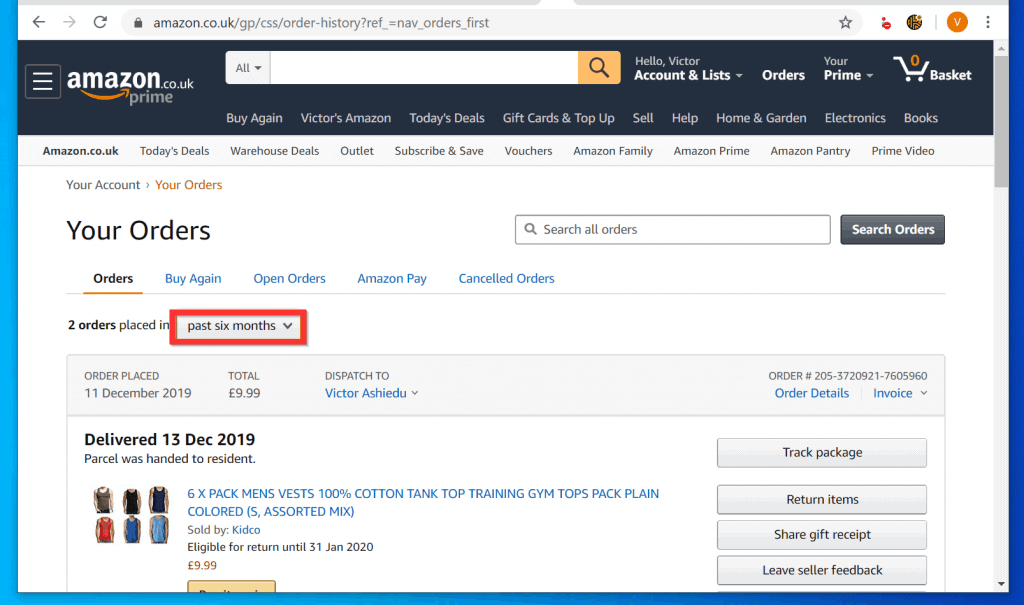Here's a cleaned-up and detailed version of the caption:

---

The image is a screenshot from an Amazon UK web page, specifically the order history section. At the top of the page, within a gray border, there are navigation options including back, forward, and refresh buttons. The URL displayed reads "amazon.co.uk/gp/css/order-history."

In the upper right corner, a profile icon enclosed in an orange circle is visible. Below this, the Amazon UK logo is prominently displayed, featuring "amazon.co.uk" with the classic orange arrow-smile logo. 

The search bar is positioned centrally and labeled "All," highlighted by an orange search indicator. Just beneath the search bar are links with text that reads: "Hello, Victor," followed by "Accounts & Lists," "Orders," "Your Prime," "Basket," and a list of navigation links including "Buy Again," "Victor's Amazon," "Today's Deals," "Gift Cards & Top-Up," "Sell," "Help," "Home & Garden," "Electronics," and "Books."

Further down the screenshot, an additional horizontal menu lists several more categories: "Today's Deals," "Warehouse Deals," "Outlet," "Subscribe & Save," "Vouchers," "Amazon Family," "Amazon Prime," "Amazon Pantry," and "Prime Video."

The section below displays Victor's order details, stating:

- Orders placed in the past six months.
- "Orders placed: 11 December 2019."
- "Total: £9.99."
- "Dispatch to: Victor Ashidi."
- "Order details" with a link to the invoice.
- "Delivered on: 13 December 2019."
- The parcel was handed to a restaurant.

The order comprises:
- Six times Pack Men's Vest, 100% Cotton.
- Tags such as "Running," "Training," "Gym Tops," "Plain Pack," "Plain Color," "Assorted Mix."

At the bottom of the section, there are options to track the package, return the item, share, view gift receipt, or leave seller feedback.